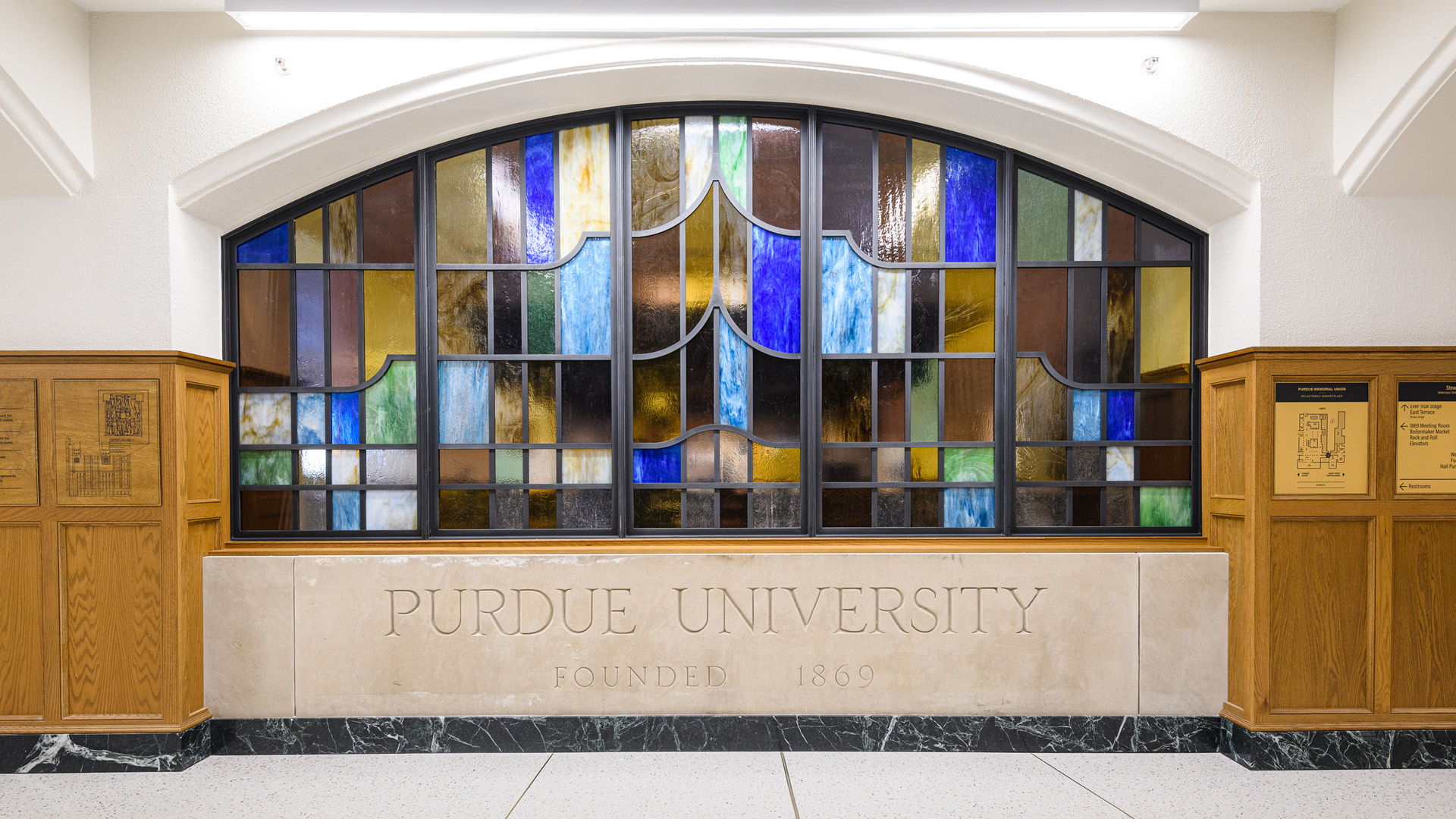The image depicts the interior of a white-painted building featuring an ornate arched window with stained glass panes in varying shades of blue, light blue, brown, and green. The window's panes are irregular rectangles and geometric shapes. Below the window, a marble-like structure is inscribed with the words "Purdue University" and "Founded in 1869." Flanking the inscription, there are two brown wooden shelves, devoid of drawers, which might function more like stands or cabinets. At the top of the image, a white light is switched on, illuminating the scene. The floor is a white tile complemented by dark marble wainscoting, adding to the room's architectural elegance.